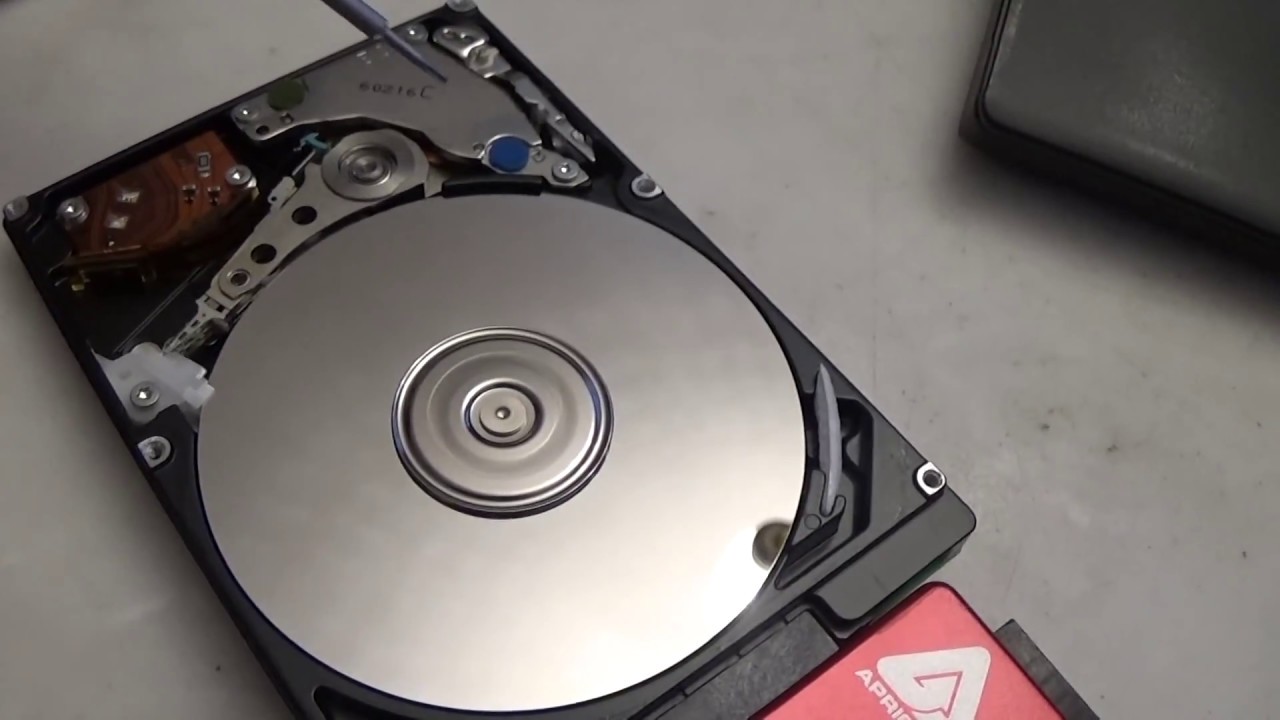The full-color image depicts the extracted disc tray of a laptop or PC, showcasing an elaborate interior, predominantly plastic and metal. Central to the image is a large, silver circular area, indicative of where a CD would be placed. This disc is encased in black plastic that houses various components. The upper-left portion of the circle features a rotating arm, leaning into the central disc. Adjacent to this, in the lower-left corner, a brown rectangular component, possibly a battery, is visible. A red segment with the letters "A-P-R-I" partially obstructed indicates some branding, positioned near the bottom right. The upper right corner includes an encroaching black box, possibly part of a laptop from which the tray was removed, adding context to the workspace. A fine-tuned screwdriver appears to be poised for maintenance or adjustments, suggesting active work on the device. The scene is set on a gray countertop with a slight view of a laptop's corner, emphasizing the technological setting.